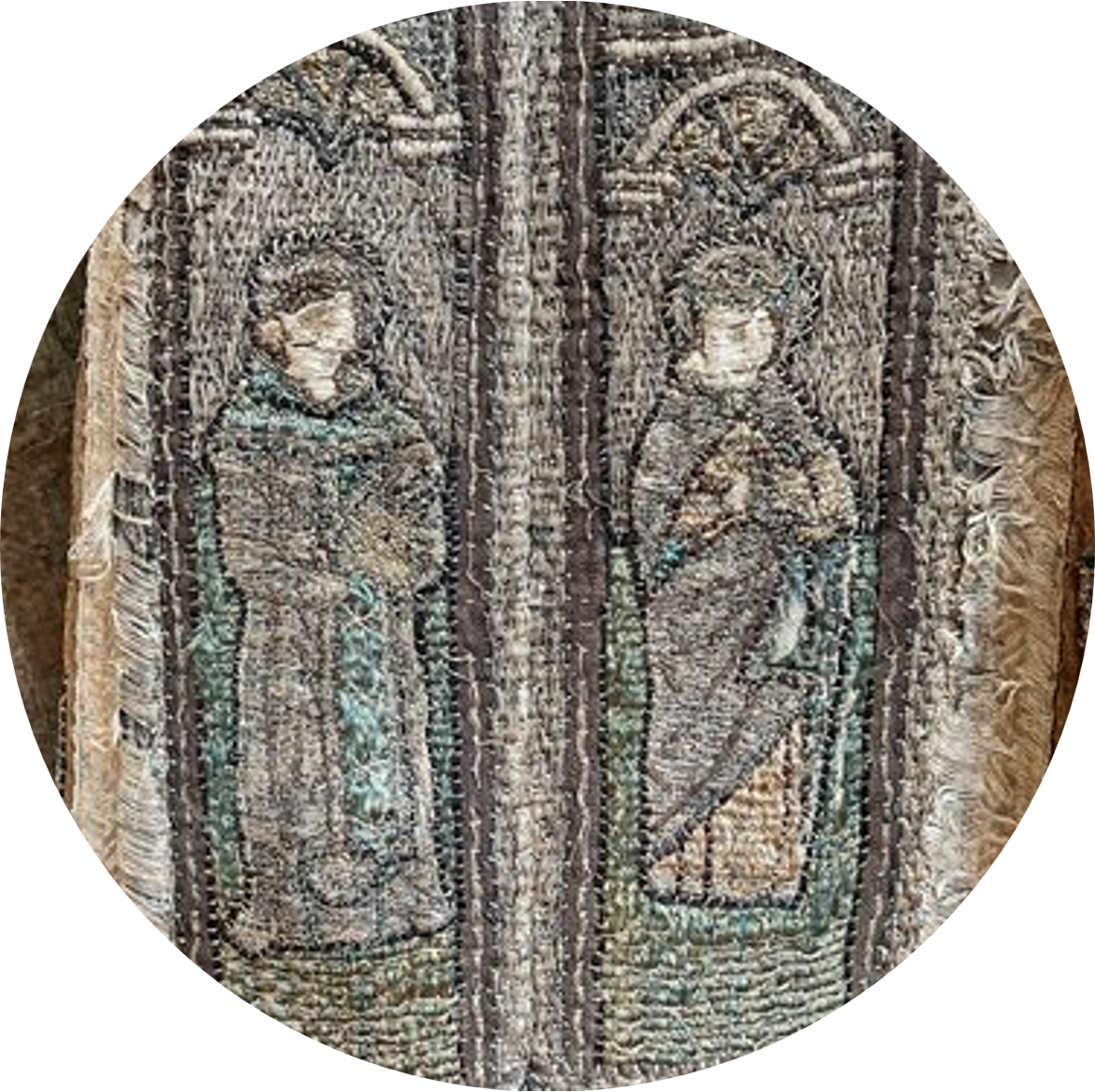This is a close-up circular photograph of an old, threadbare tapestry showcasing intricate hand-sewn details that reflect its considerable age. The tapestry features two religious figures, likely monks or saints, each occupying a separate panel divided by a vertical line. Both figures are depicted with halos behind their heads and are clad in long, faded brown robes. The figure on the left is distinguished by a green scarf hanging down the middle of his body, while both figures are framed by archways over their heads. The colours of the tapestry have significantly faded over time, now presenting muted shades of green, purple, blue, gray, and occasional hints of red. This wear and passage of time are further accentuated by frayed edges where the stitching has begun to pull away. The once vibrant embroidery is now a pale echo of its former self, capturing the viewer's attention with its historical and religious significance.